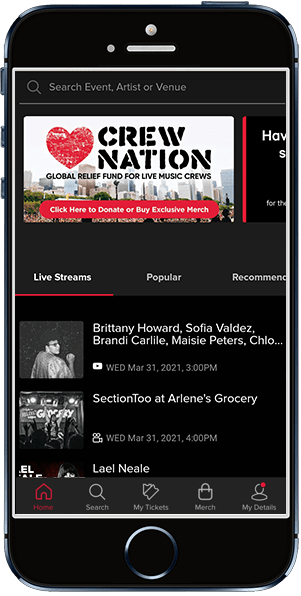The image is a detailed screenshot displayed on a black smartphone, showcasing what appears to be a video viewing app in its nighttime mode. The app interface features a search bar at the top where users can look up events, artists, or venues, suggesting it is tailored for live music streams. The main content displays a promotional banner for the "Crew Nation, Global Relief Fund for Live Music Crews," with a red call-to-action banner at the bottom urging users to "click here to donate or buy exclusive merch."

Below the banner are three navigation tabs labeled "Live Streams," "Popular," and "Recommended," with "Live Streams" currently selected, indicated by a red underline. The live stream section lists several artists, including Brittany Howard, Sophia Valdez, Brandi Carlisle, Macy Peters, and Chloe, with scheduled performances. Specifically, 'Section Two at Arlene's Grocery' has detailed scheduling information, showing performances on Wednesday, March 31st, 2021, at 3 PM and 4 PM, respectively.